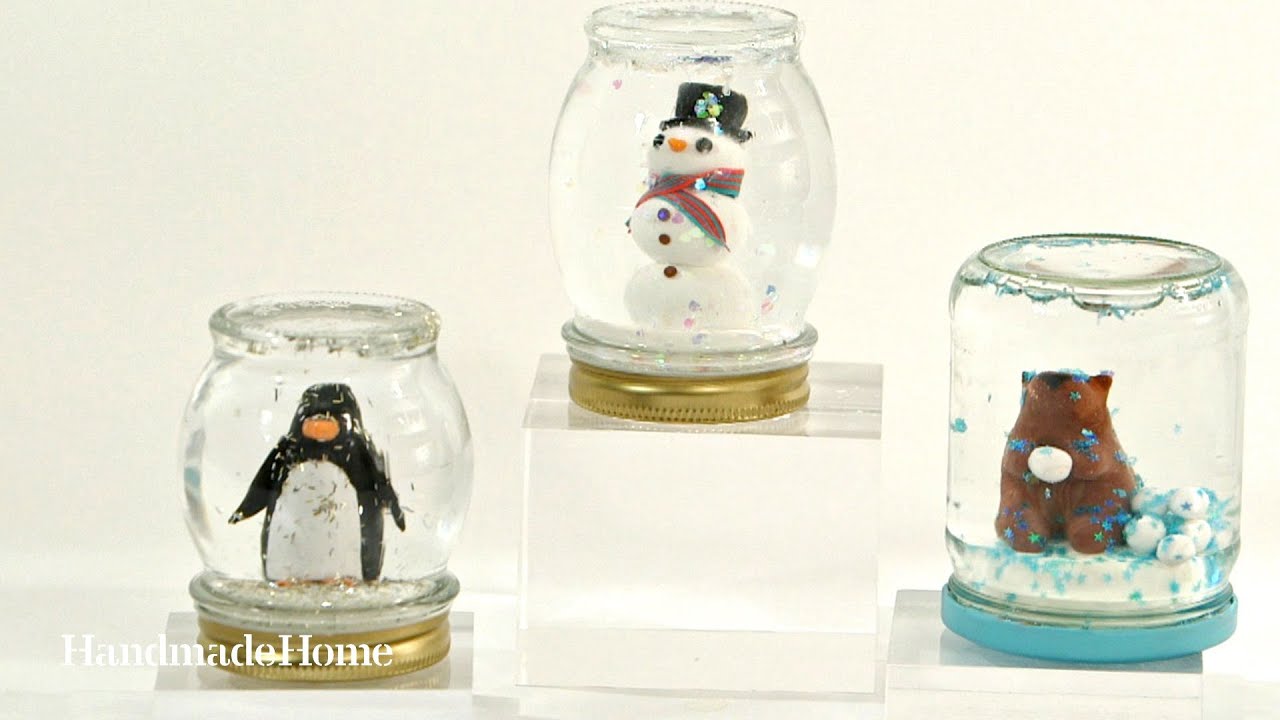The photograph showcases three charming homemade snow globes crafted from baby food jars, set against a white surface with a beige background. Each globe houses a different winter-themed figurine. The globe on the left, topped with a gold lid, contains a small penguin with a black body, white stomach, and orange beak. The central globe, elevated on a clear plastic cube and also featuring a gold lid, displays a classic snowman adorned with a black top hat, a red striped scarf, black buttons, a carrot nose, and two black eyes. The globe on the right, unique with its blue lid, holds a brown bear sitting on snow, appearing to hold a snowball with extra snowballs around it. A white text overlay at the bottom left corner reads "handmade at home," indicating this adorable craft project, likely sourced from a crafting site, offers a budget-friendly and enjoyable activity for children.